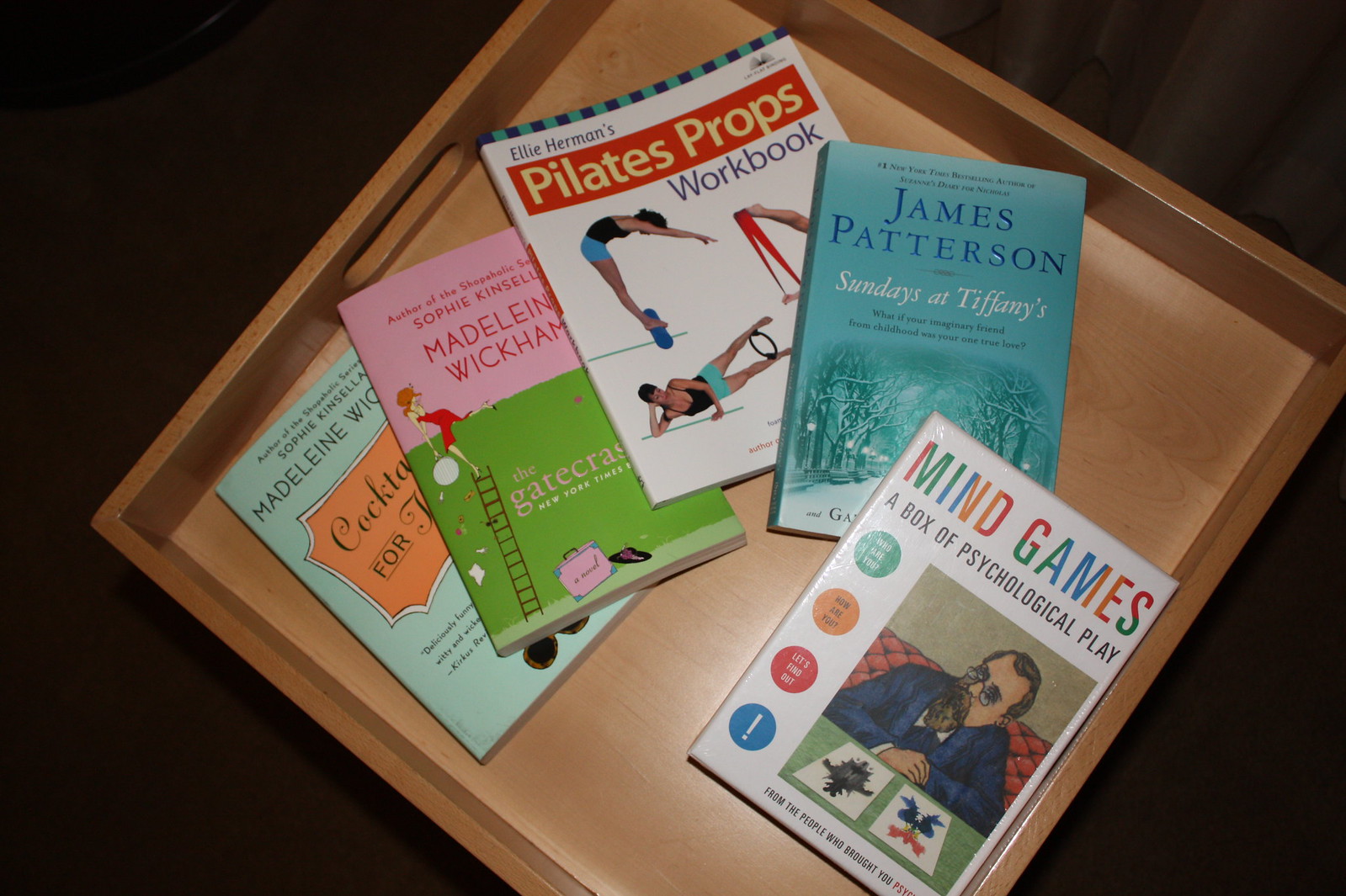The photograph displays a wooden pull-out bin angled diagonally, forming a diamond shape against an entirely black background. The handle is visible in the upper left corner. Inside the bin are five books of various colors and sizes, stacked somewhat haphazardly. 

The bottom book is light blue with an orange title, possibly a Sophie Kinsella paperback. Above it is a book with pink and green on its cover, its details obscured. Next is "Ellie Herman's Pilates Props Workbook," which features a woman performing Pilates and is primarily white with a red-highlighted title. Above this is James Patterson's "Sundays at Tiffany's," characterized by its blue cover. The top book, "Mind Games," has a white cover with an illustration of a man looking at inkblots, and colorful letters in the title. The books appear in no specific order, each adding a splash of color to the scene within the rustic brown wooden bin.